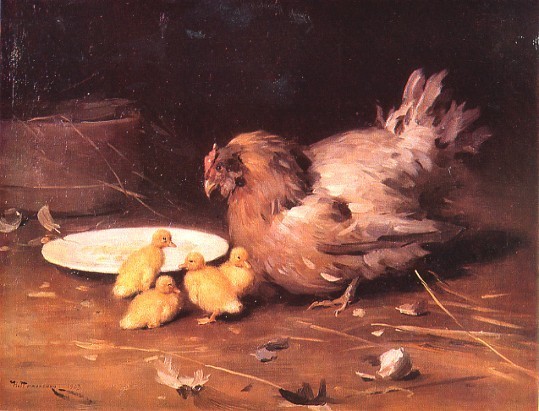The image is a detailed hand-painted artwork depicting a serene farmyard scene. In the center, it showcases a large rooster, predominantly grayish with red comb, brown breast, and shoulders. Surrounding the rooster on the right are four yellow chicks, with one sitting and the other three standing. The chicks’ innocent curiosity is evident as they look in various directions. Behind them, there is a white plate, likely a dish for food. The ground is a hard, brown flooring scattered with straw, hay, leaves, and feathers, adding to the rustic charm. In the top left corner, a bucket can be discerned, contributing to the farmyard setting. The overall coloration includes black, gray, brown, white, yellow, and tan, which enhances the natural, earthy feel of the painting. The absence of text directs full attention to the detailed artwork.